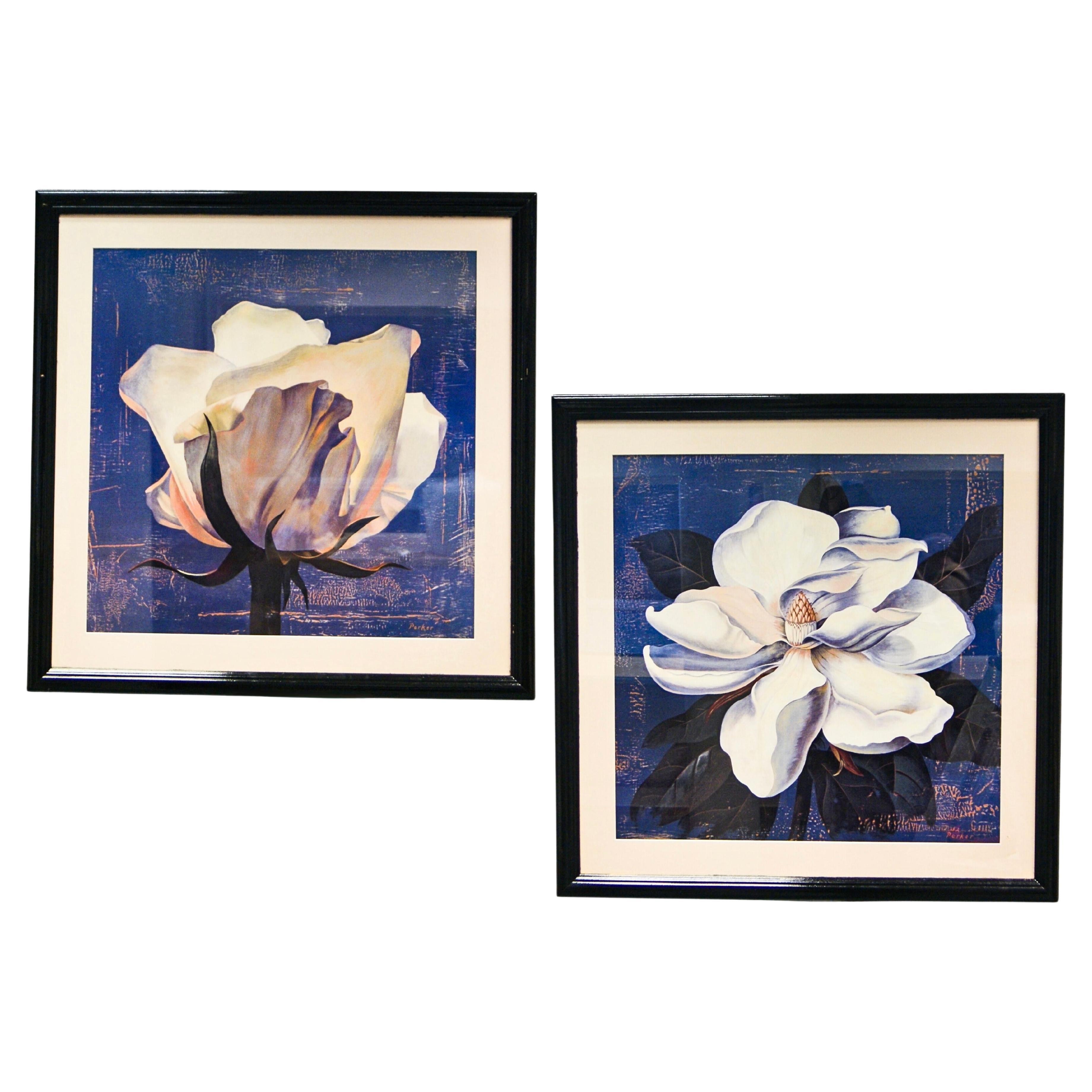The image displays two framed watercolor paintings of white flowers set against a white backdrop. Both paintings are positioned slightly wider rather than taller; one in the upper left and the other in the lower right of the frame. 

The upper left painting features a side view of a white flower with purple accents, prominently centered and surrounded by a blue background. The lower right painting offers a top-down perspective of a white flower, complemented by green leaves and a similar blue background. Both pieces emphasize the delicate details of the flowers, showcasing the elegance of watercolor techniques.